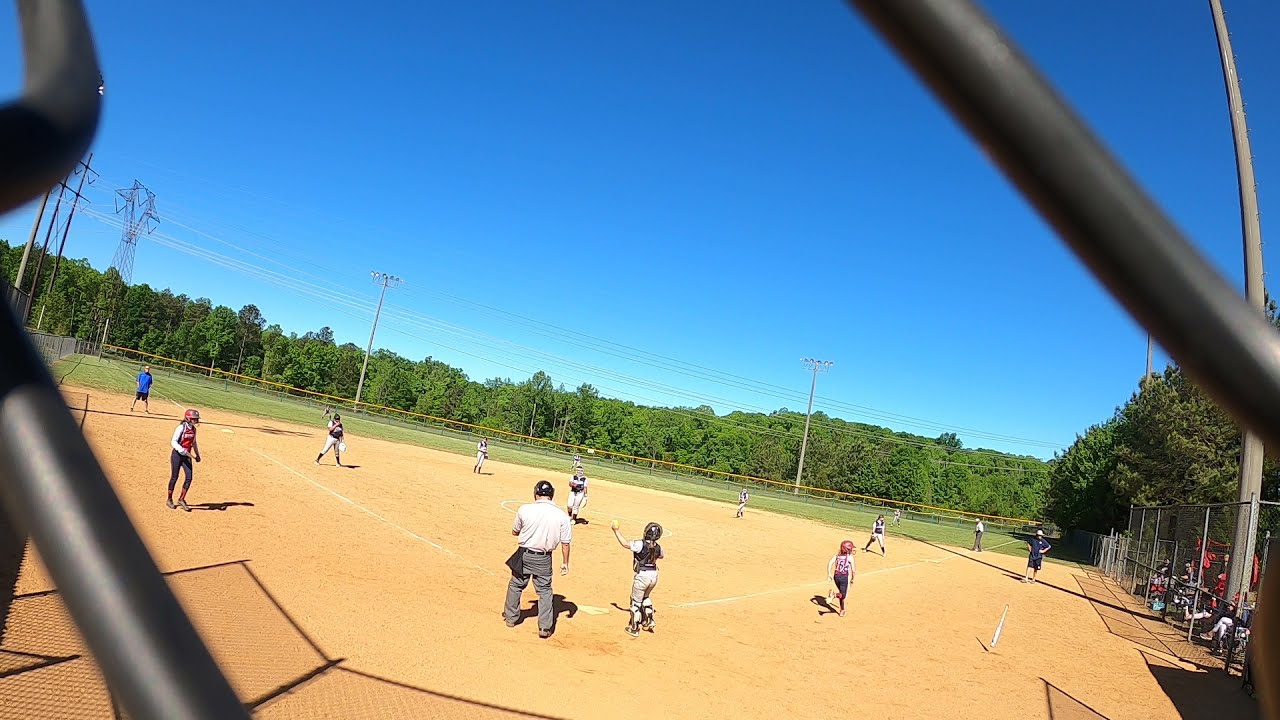The image is a color photograph in landscape orientation, capturing a lively scene of a little league baseball game. The picture appears to have been taken through a chain-link fence, which borders the frame in an extreme close-up, suggesting the viewer's presence close to the action, likely near home plate. The field is a red-dirt baseball diamond set in a local park, with green grass outfield encircled by fencing topped with yellow trim. Beyond the fence, stadium lighting and large power lines stand against a backdrop of densely populated trees under a clear, blue midday sky.

In the foreground, a young player at bat is caught mid-action, wearing a helmet, a white shirt, and gray pants, and is seen holding his left hand up. A bat is visible midair to the right, indicating a recent hit. Another player, possibly the catcher, seems poised to throw the ball towards the pitcher. An umpire, dressed in green pants and a white shirt with a black face mask, stands behind the batter. The photo captures the hustle and energy typical of little league games, with players running to their next bases and fielders in their positions, all set against the vibrant outdoor setting.